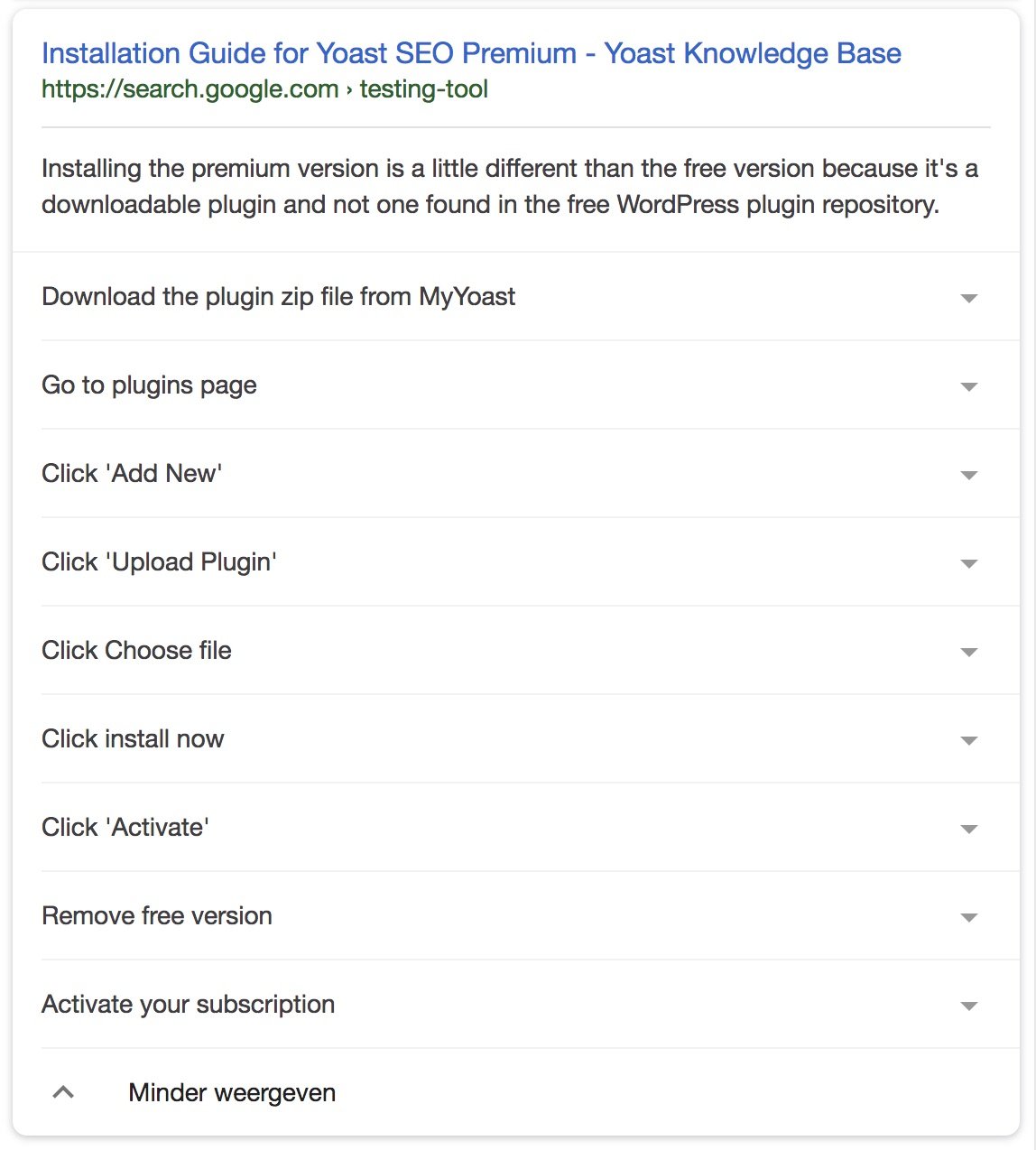**Descriptive Caption:**

The image shows a Google search result page focused on installing the Yoast SEO Premium plugin. 

At the top, highlighted in blue text, is the title: "Installation guide for Yoast SEO Premium - Yoast Knowledge Base." Directly below the title, the URL is displayed as "https://searchgoogle.com/testmethod."

The search snippet in black text explains that installing the premium version of Yoast differs from the free version, emphasizing that it is a downloadable plugin, unavailable in the free WordPress plugin repository.

Below this explanation is a vertical list of steps required for installation, each accompanied by a right-aligned, clickable drop-down arrow to reveal more details. The steps are as follows:
1. Download the plugin zip file from My Yoast.
2. Go to the Plugins page.
3. Click 'Add New.'
4. Click 'Upload Plugin.'
5. Click 'Choose File.'
6. Click 'Install Now.'
7. Click 'Activate.'
8. Remove the free version.
9. Activate your subscription.

At the very bottom of the list, an upward-facing arrow is present next to the phrase "Mender with Grieving," which does not have a drop-down option.